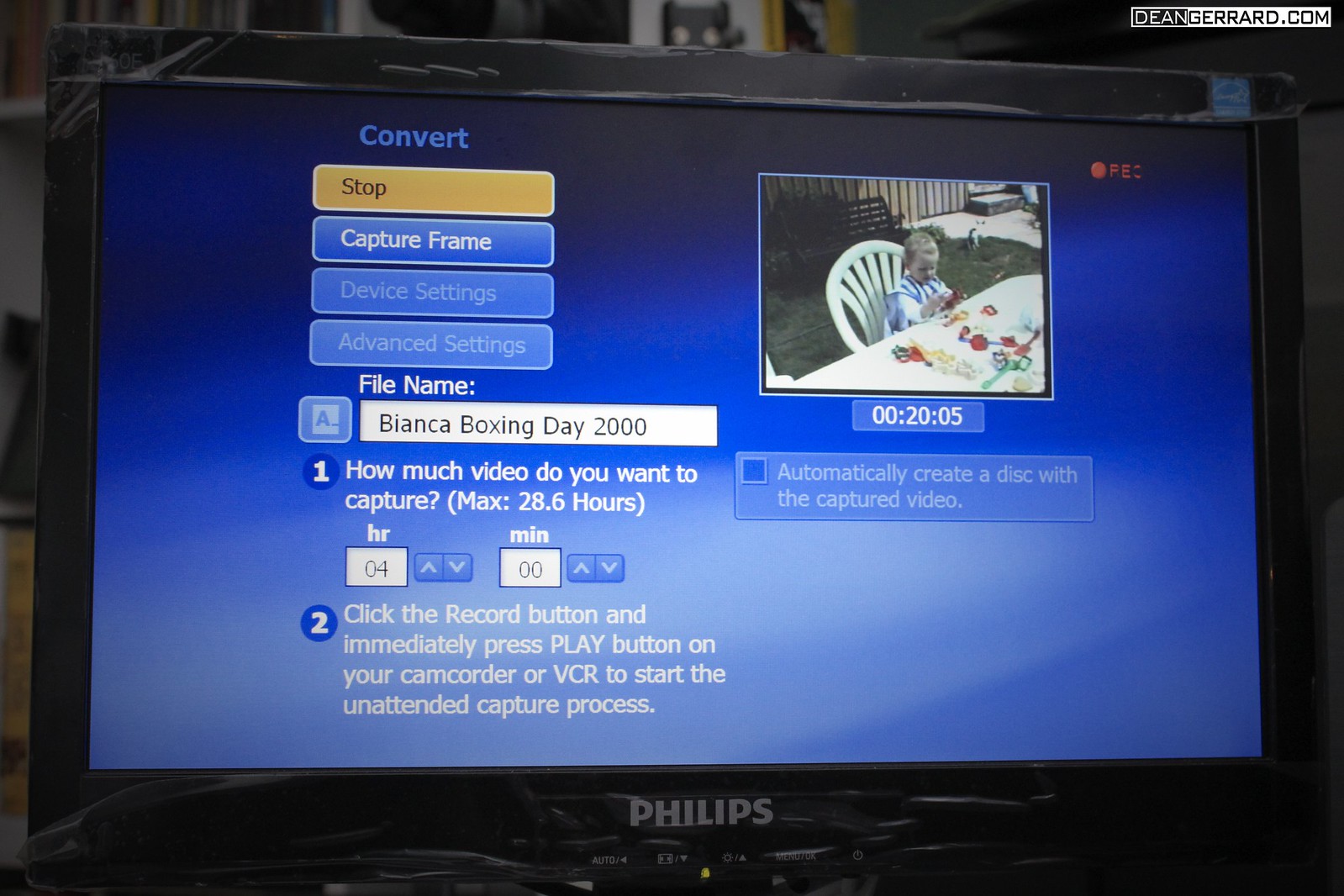This close-up photograph features a Philips TV screen occupying the central focus, framed by a black border. The image background is slightly blurred, indicating an indoor setting, possibly a personal computer room. The TV screen displays a blue menu interface with several options listed on the left-hand side: "convert" at the top, followed by buttons labeled "stop" (in yellow), "capture frame" (in dark blue), "device settings," and "advanced settings." Below these, a white text bar reads "File name: Bianca Boxing Day 2000" (2018 in another account), and beneath that, instructions for video capture, stating, "How much video do you want to capture? Max 28.6 hours," with four hours selected via up and down arrow controls. Another section instructs, "Click the record button and immediately press play on your camcorder or VCR to start the unattended capture process."

In the upper right corner of the screen, a small thumbnail depicts a child seated at a table, engaged in a colorful activity, with a 00:20:05 timestamp and a blinking "REC" recording logo, indicating a live capture. At the bottom of this thumbnail, text mentions, "automatically create a disk with captured video." The image is topped off with a watermark outside the TV screen on the upper right, bearing the logo "DeanGerard.com." The visual amalgamation of these details presents a vivid snapshot of a video-capturing setup in progress.